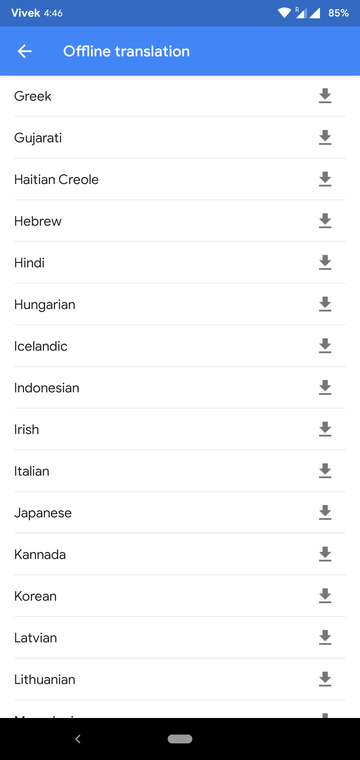This image captures a segment of a mobile application, specifically the offline translation settings page, likely on a device named "Vivek." The time displayed is 4:46, with full Wi-Fi bars and an 85% battery level. At the top, "Offline Translation" is highlighted in blue, accompanied by a left arrow for navigation back to previous settings. 

The visible portion of the list showcases 15 languages available for offline translation, sorted alphabetically, suggesting the list extends both upwards and downwards beyond the current view. The languages displayed include Greek, Gujarati, Haitian Creole, Hebrew, Hindi, Hungarian, Icelandic, Indonesian, Irish, Italian, Japanese, Kannada, Korean, Latvian, and Lithuanian. This partial list indicates the user was likely scrolling through available options before pausing to capture this screenshot.